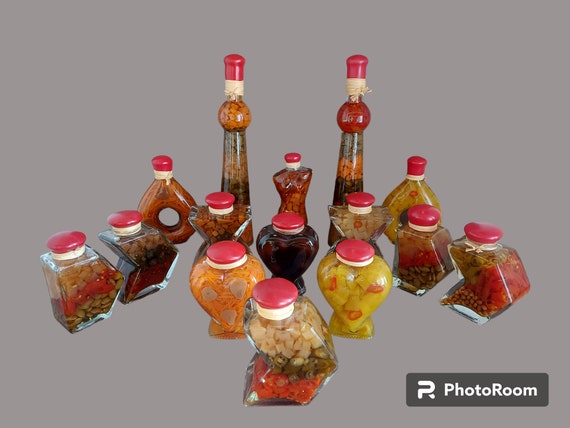The rectangular image showcases approximately 14-15 glass bottles of different sizes and shapes, all filled with what appears to be pickled vegetables, resting against a plain gray background. The bottles exhibit a variety of designs, including tall, cylindrical, angular, and curvilinear forms, all capped with distinctive round red lids. Vegetables such as carrots, beans, and sliced peppers—including jalapenos—are prominently visible through the transparent glass. Some bottles also contain mixed or singular varieties of beans in hues of red, green, black, and orange. A detail that stands out includes a darker-colored bottle centrally located among the others. Below the display, a small, dark gray rectangle with beveled edges houses the text "Photo Room" in white print with a large 'R' on the left side.